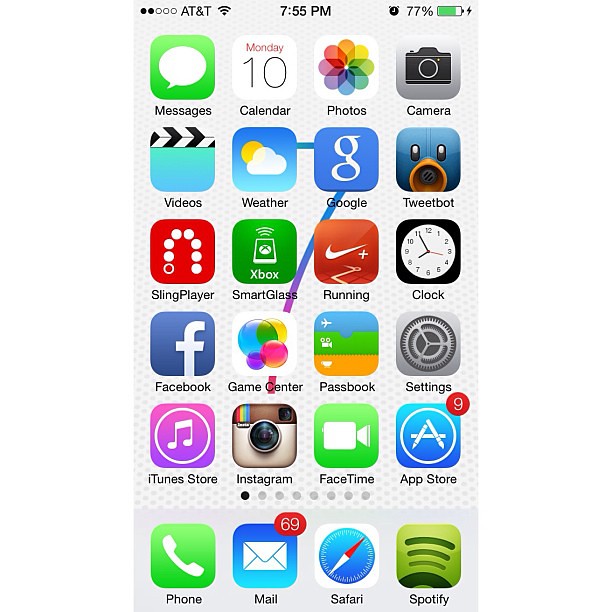The image showcases a smartphone screen, specifically an iPhone, with a rather plain background of gray polka dots on a white base. At the top of the screen, the status bar indicates the device is connected to the AT&T network, with a Wi-Fi symbol, the time displayed as 7:55 PM, and the battery level at 77%—evidenced by the mostly green battery icon.

The home screen displays five rows of apps, totaling 20 icons visible on this page alone, with more apps likely present on additional screens. The first row of apps includes the Messages app (depicted by a white speech bubble on a green background), Calendar (showing today's date as 'Monday the 10th'), Photos (characterized by a multicolored flower made of overlapping circles), and Camera (marked by a camera icon).

The second row features the Videos app, followed by Weather (symbolized by a cloud and sun graphic), Google (with its classic lowercase 'g' on a blue background), and Tweetbot (featuring a quirky bluebird visage with an open beak).

In the third row, the Slingplayer app has an icon that resembles a dental mold or bite mark. It's followed by the SmartGlass app for Xbox, displaying a tiny controller logo, the Nike Running app (illustrated with a swoosh and a road meandering into the horizon), and the Clock app (represented by a clock face).

The fourth row contains Facebook (with its distinct 'f' on a blue background), Game Center (depicted by colorful bubbles), Passbook (showing various icons including an airplane), and Settings (featuring a nested gear or sprocket graphic).

The last visible row includes the iTunes Store (with a musical note on a purple background), Instagram (showing its well-known camera logo), FaceTime (having a white camcorder icon on a green background), the App Store (accompanied by a notification badge displaying the number 9), and finally the Phone app.

At the bottom, the persistent dock displays four more built-in apps: Phone, Mail (noting 69 unread messages), Safari (illustrated by a compass icon), and Spotify.